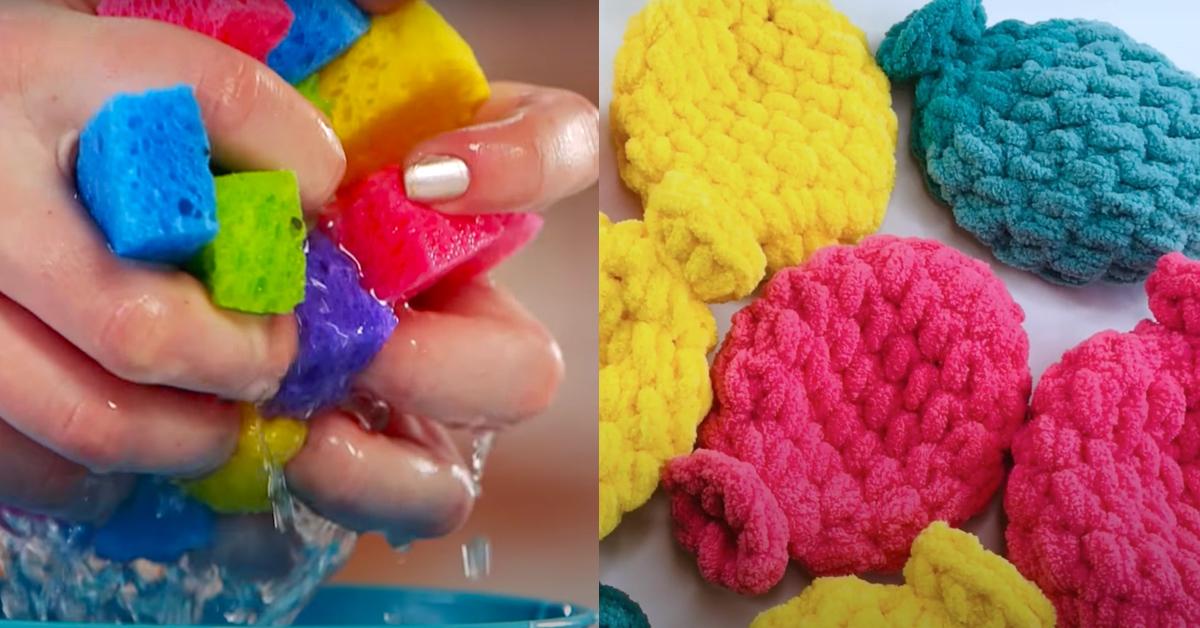The image displays two side-by-side photographs, each capturing sensory materials used in occupational therapy. The left photograph is a close-up shot focusing on hands squeezing a collection of water-soaked sponges, dripping water as they are compressed. There are multiple sponges visible: blue, yellow, reddish-pink, dark indigo, and a second reddish-pink sponge. The visible part of the person’s hand features a shiny silver nail polish on the left forefinger, adding a touch of metallic sparkle. The right photograph presents several knitted balloon-like objects, arranged side-by-side. These deflated whoopee cushion-shaped items exhibit a vibrant array of colors: two yellow on the left, one bluish-green at the top right, two pink at the bottom right, and a partly visible yellow one peeking into the frame. These colorful knitted pieces, made of fuzzy yarn, echo the bright hues of the sponges and are used as sensory stimulation tools in therapy sessions, akin to the tactile experience provided by the sponges.